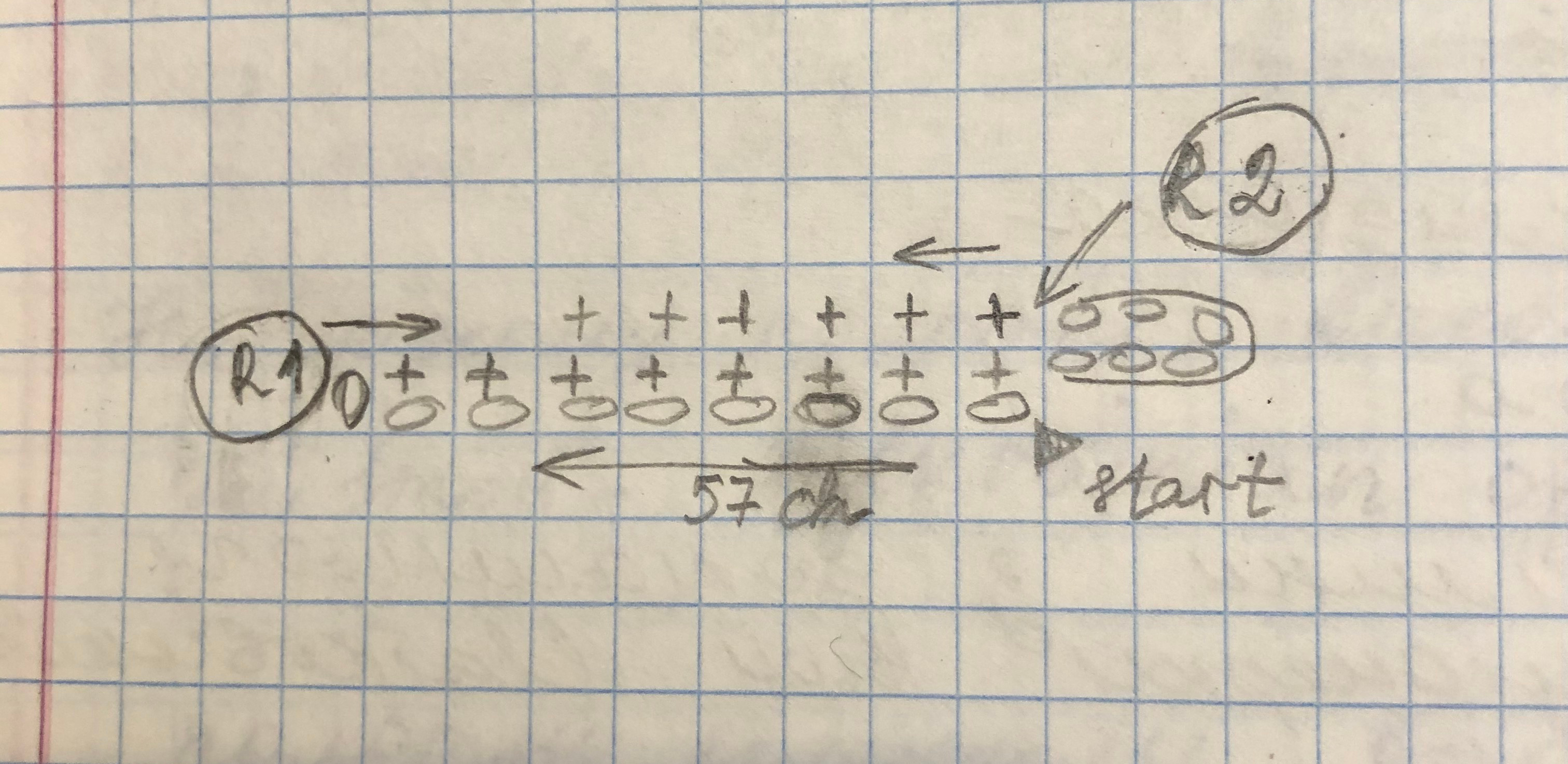This detailed image features a sheet of grid paper that appears to come from the later portion of a notebook, indicated by a pink line running down the left-hand side, characteristic of certain notebooks' margins. The grid is formed by evenly spaced blue lines creating small squares. 

Upon closer inspection, the reverse side of the paper reveals imprints of text, likely written with a firm hand using a pencil, suggesting active use of the page on the flip side.

The primary focus of the content on this page appears to be a complex diagram involving several circles, arrows, and cross marks that resemble a mathematical or logical flowchart. On the left, there is a circle labeled "R1" with an arrow pointing to the right at its top edge. Additionally, below this primary circle, there are nine smaller circles arranged in a vertical line. The first small circle is plain, while the remaining eight have crosses above them. In the row aligned with the arrow extending from the "R1" circle, every fourth cube in the grid features a cross mark.

Towards the right-hand side of the page, there is another set of circles. At the top, there are three circles aligned vertically, with a subsequent line of three circles positioned below them. Above these circles is another circle labeled "R2," with an arrow pointing downward towards the row with the first set of crosses. Additionally, an arrow extends from the "R2" circle back to the left.

At the bottom of the diagram, the word "start" appears, accompanied by an arrow pointing to the right. Overlaying these elements is a large, horizontal arrow running from left to right across the diagrams of circles and crosses, labeled "57 CH."

This diagram seems to represent a procedural or algorithmic path, though its full context and specific meaning are not immediately clear.